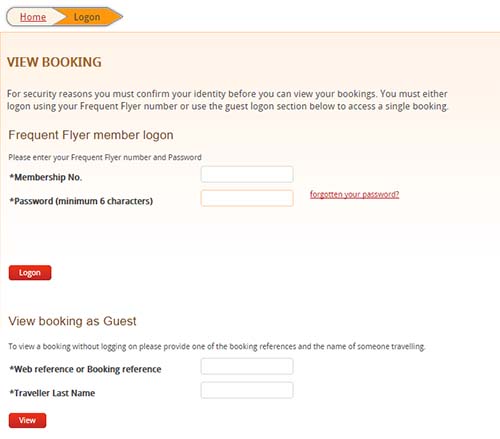The image depicts a user interface element that resembles a pencil shape divided into two sections. The lower portion is a cream color tapering to a point, featuring the word "Home" in red, underlined. The upper section is orange and also tapers to a point, displaying the text "Log On".

Below these sections, there is an orange rectangle that gradually fades to a lighter orange towards the bottom, containing the text "View Booking" in brown. Underneath this are some black words that are too small to decipher. The phrase "Frequent Flyer Member Log On" appears, followed by text that is illegible due to its small size.

Two sections, marked with stars, indicate fields for "Membership No." and "Password" (with a note specifying a minimum of six characters). To the right of the "Membership No." field is a white rectangle outlined in gray, while below this is another similarly outlined white rectangle.

Further to the right is red text, followed by a red rectangle labeled "Log On". Below this, the text "View Booking as Guest" appears, accompanied by more small, unreadable text. The image also includes fields for "Web Reference or Booking Reference" and "Traveler Last Name", each indicated by a star and accompanied by gray-outlined white rectangles. At the bottom of the composition, a red rectangle contains the text "View".